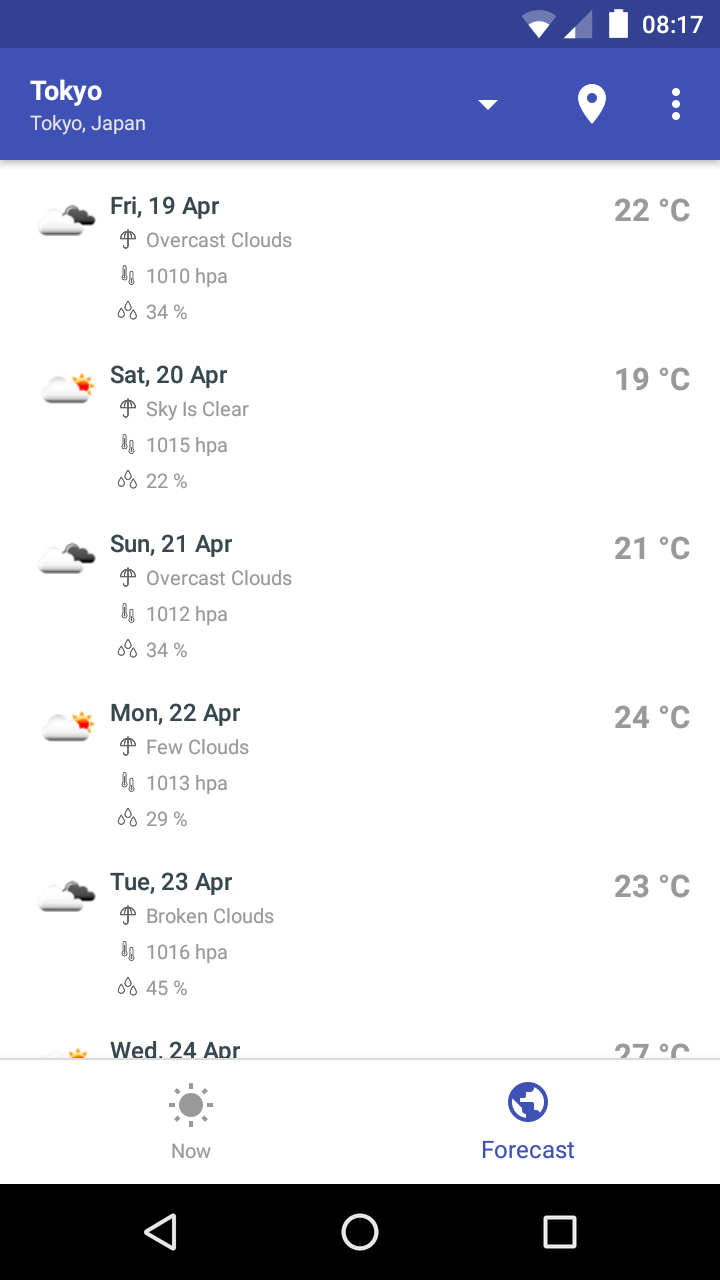In the screenshot from a cell phone, a weather forecast app is open. At the top-right corner, the status bar displays several icons: the Wi-Fi signal, the cell phone signal strength, and the battery level, which shows a time of 1:17. Below this, to the left, the app indicates the current city as "Tokyo," with a subsequent line clarifying "Tokyo, Japan." To the right in the same bar, there is a drop-down arrow, a GPS pin icon shaped like a teardrop, and a vertical ellipsis (three vertically aligned dots).

Below this bar, the screen shows detailed weather information for two days. For Friday, April 19th, the weather is reported as 22 degrees Celsius with overcast clouds, a pressure of 1010 hPa, and a 34% chance of rain. For Saturday, April 20th, the forecast predicts a clear sky with a temperature of 19 degrees Celsius, a pressure of 1050 hPa, and a 22% chance of rain.